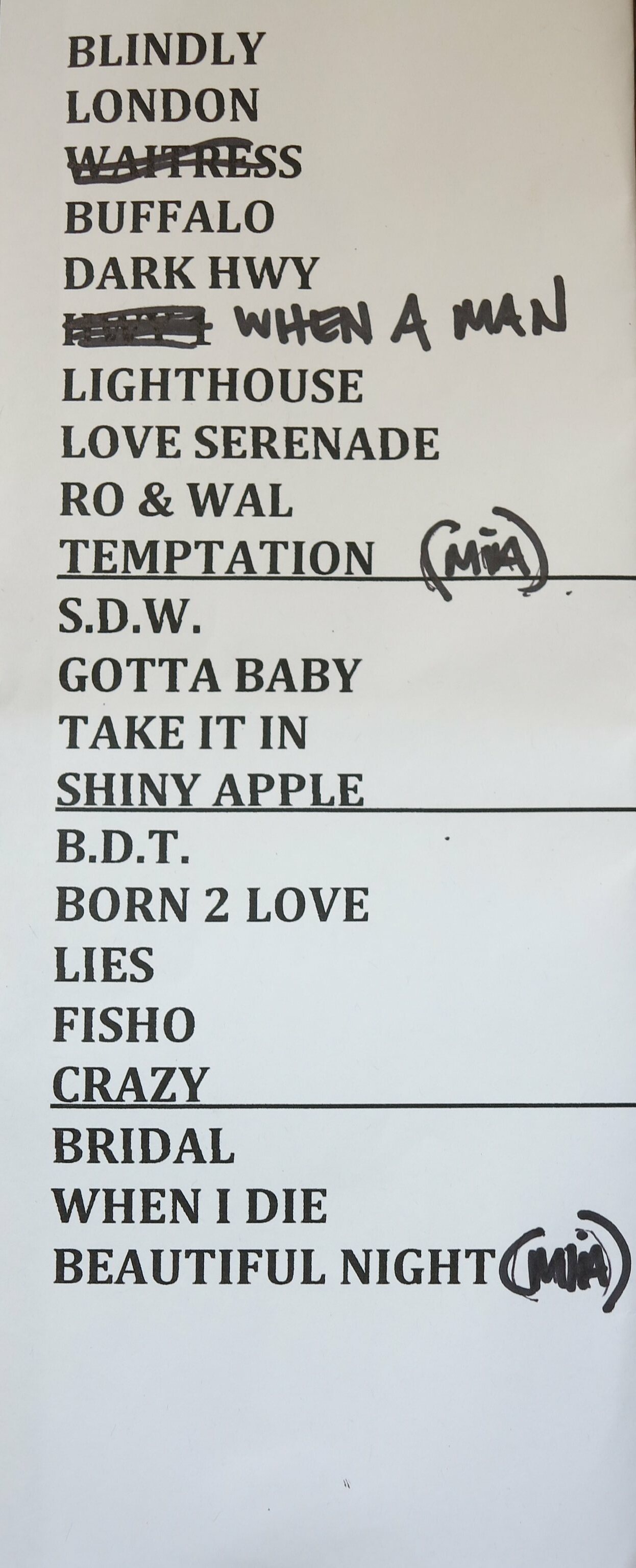The image depicts a grayscale typed list on a grey background, with the text in black. At the top in bold capital letters is "BLINDLY," followed by "LONDON." The next entry, "WAITRESS," is crossed out with a curved line from the bottom of the 'W' to the 'E'. Following this are "BUFFALO," "DARK HIGHWAY," and another indiscernible crossed-out word. Next is "WHEN A MAN," followed by "LIGHTHOUSE," "LOVE SERENADE," "ROW AND WALL," and "TEMPTATION" with "MIA" written in parentheses. Below a black line is "SDW," succeeded by "GOTTA BABY," "TAKE IT IN," "SHINY APPLE," and "BDT." The list continues with "BORN TO LOVE," "LIES," "FISHO," "CRAZY," and "BRIDAL." Finally, it concludes with "WHEN I DIE" and "BEAUTIFUL NIGHT," with "MIA" noted again in parentheses. The organization of the terms, some underlined and others struck out, suggests a structured playlist or list of titles.